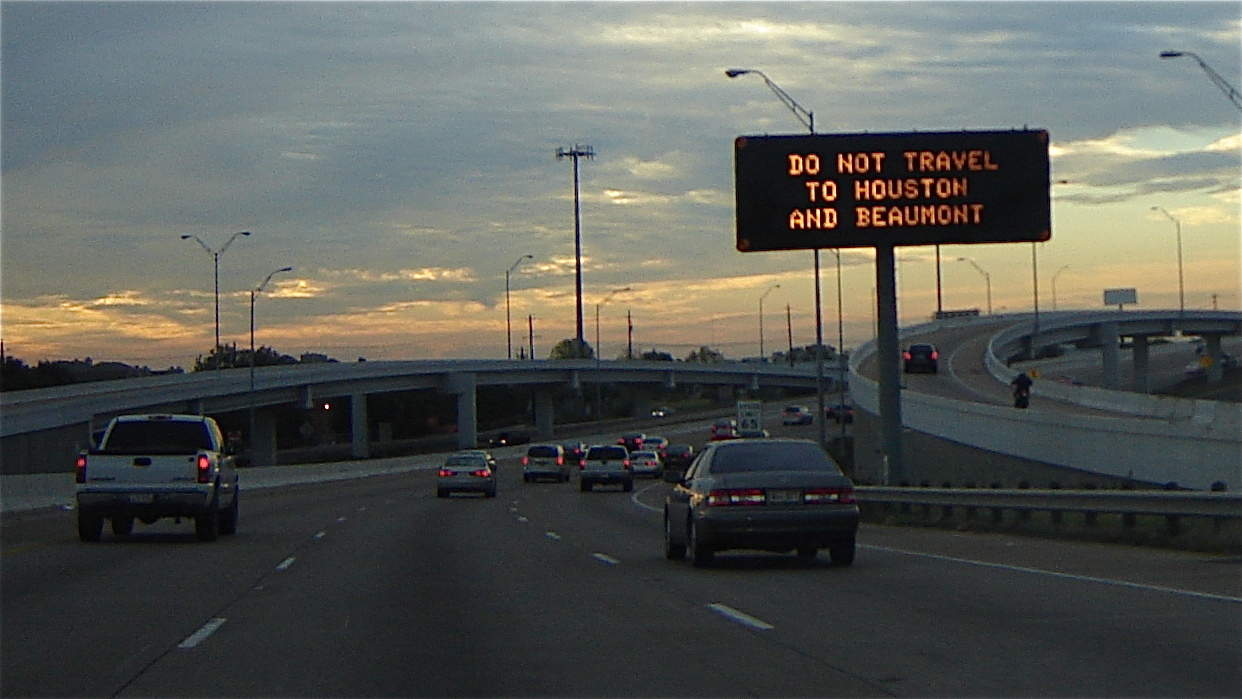This detailed outdoor photograph, likely taken at either dusk or dawn, captures a realistic highway scene under a partly cloudy sky. The horizon reveals a blend of light blue with streaks of red and yellow, suggesting the sun is either rising or setting. In the foreground, a three-lane highway stretches out, with dark pavement and dotted white lane markings. To the left, an overpass can be seen along with green trees in the background. On the right side of the image, an on-ramp curves towards the center before veering back to the right.

Centered in the image are the rears of approximately 10 to 15 vehicles, including white pickup trucks, gray sedans, and various other light-colored cars, all with noticeable red taillights. A tall pole on the right supports a large, rectangular digital sign in yellow-orange text on a black background, which reads, “Do not travel to Houston and Beaumont.” Additional elements in the image include various poles, a traffic light, and a tall cell tower scattered around the highway. The overall tone of the image is calm yet foreboding, with the embedded message warning against travel.